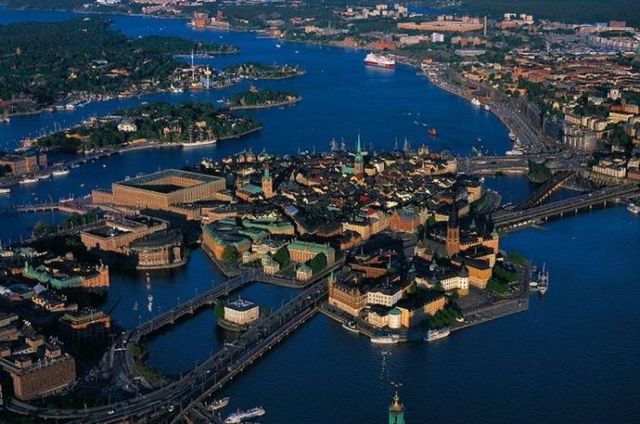This captivating aerial view showcases an unidentified European city situated on a picturesque coastal region. The cityscape is characterized by a sprawling, relatively low-density collection of buildings that line the shores and extend inland. Nestled along an intricate network of waterways and small landmasses, the area appears to be part of a shoreline inlet where freshwater and saltwater might intermingle. The interconnected islands are linked by a series of highways, creating a stunning visual of urban development intertwined with natural aquatic formations. The water is a striking, vivid blue, adding to the overall charm and beauty of the scene.